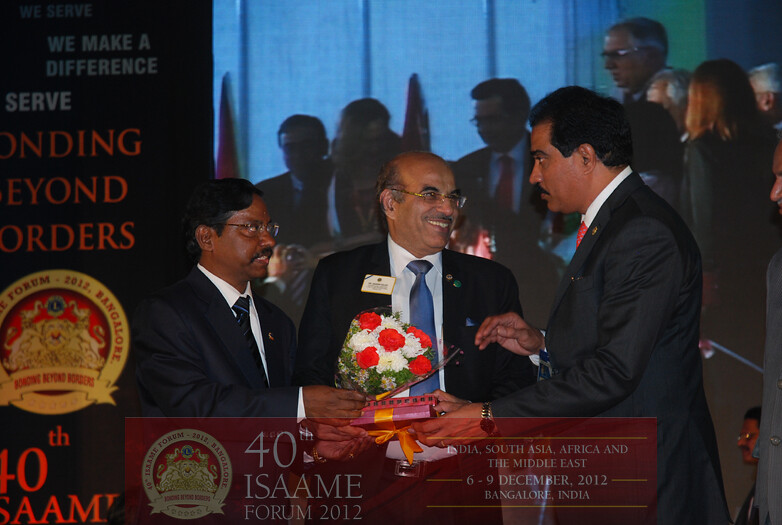In the photograph, three men are positioned on a stage during an award ceremony, likely the 40th ISAAME Forum 2012, held from December 6-9 in Bangalore, India. They appear to be of Indian origin, all dressed in black suits and ties, with dark hair and glasses. The man in the middle has a receding hairline, thin clear-rimmed glasses, a bit of a mustache, and wears a black suit with a blue tie. He is smiling at the man on the right while holding a bunch of red and white flowers and a pink-wrapped gift box with an orange ribbon and bow. The tallest man on the right, with thick black hair and a black suit with a red tie, is looking at the middle man, with one hand reaching towards the flowers or the gift. The shortest man on the left, also with dark skin, glasses, a beard, and thick black hair, appears to be presenting or sharing the gift. Behind them, a large screen displays a projected image of other people at the event. To the left of the image, a partially visible black banner reads “We serve, we make a difference,” along with references to the 40th ISAAME Forum.